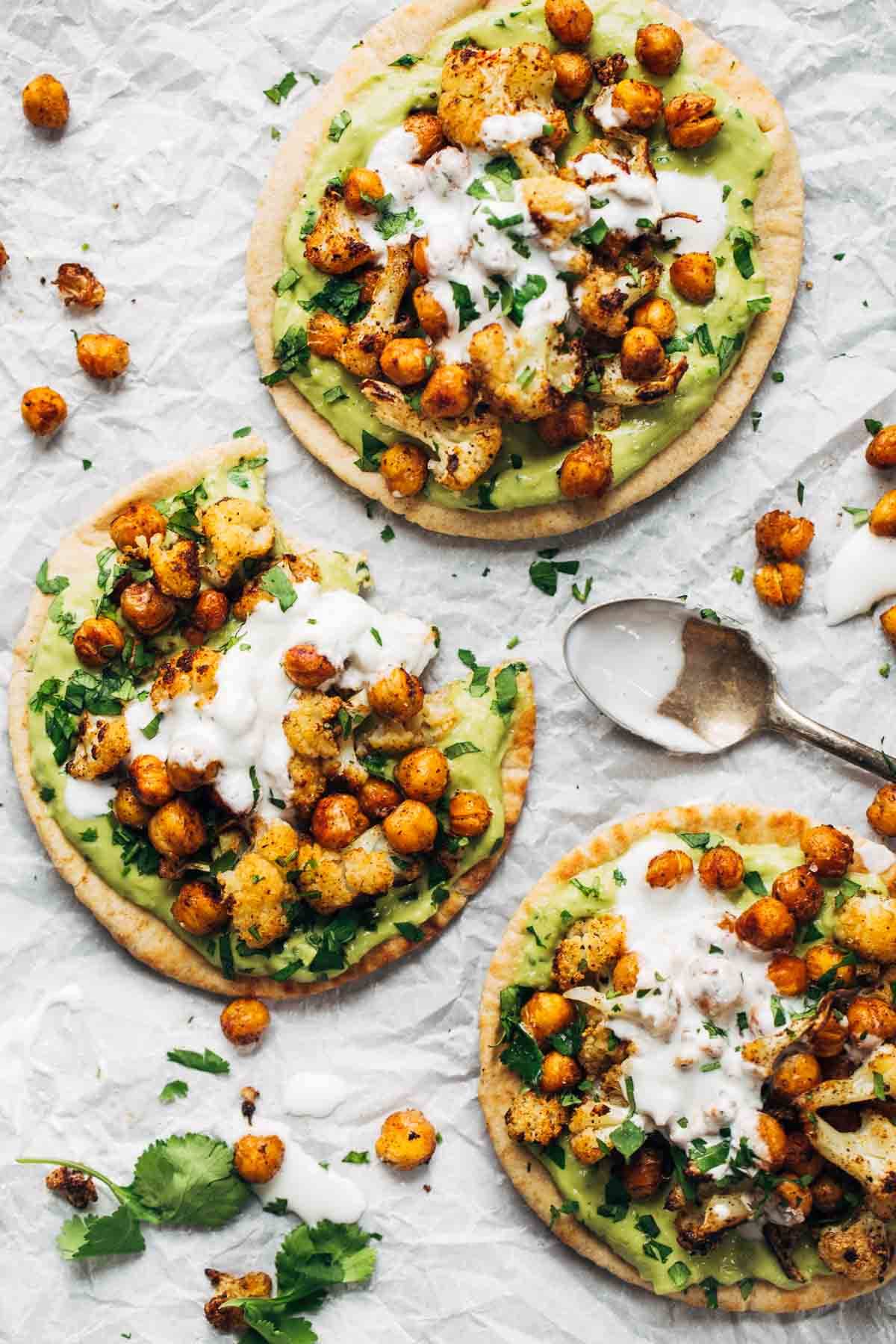This image, likely taken for a cooking magazine or online article, depicts a meticulously arranged kitchen scene showcasing a delectable dish. The photograph features three tortillas, or possibly naan breads, laid out on a light-colored, crinkled paper sheet that serves as a rustic table setting. These flatbreads are generously topped with a creamy avocado spread, succulent pieces of chicken, cauliflower, chickpeas, and a drizzle of a white sauce, likely sour cream. Garnishing the dish are finely chopped parsley and a few scattered chives, adding a burst of color and freshness.

Positioned in a triangular formation, one tortilla sits at the top right, another towards the middle left, and the third at the bottom right. Notably, the tortilla in the center has a couple of bites taken out, adding a touch of casual realism to the presentation. Chickpeas are dispersed around the tortillas, with some located at the top left, middle right, and bottom left of the image. A spoon, likely used to dollop the white sauce, rests on the crinkled paper, enhancing the sense of a recently prepared meal. This visually appealing and detailed setup undoubtedly aims to entice viewers, showcasing the dish's texture and vibrant ingredients.